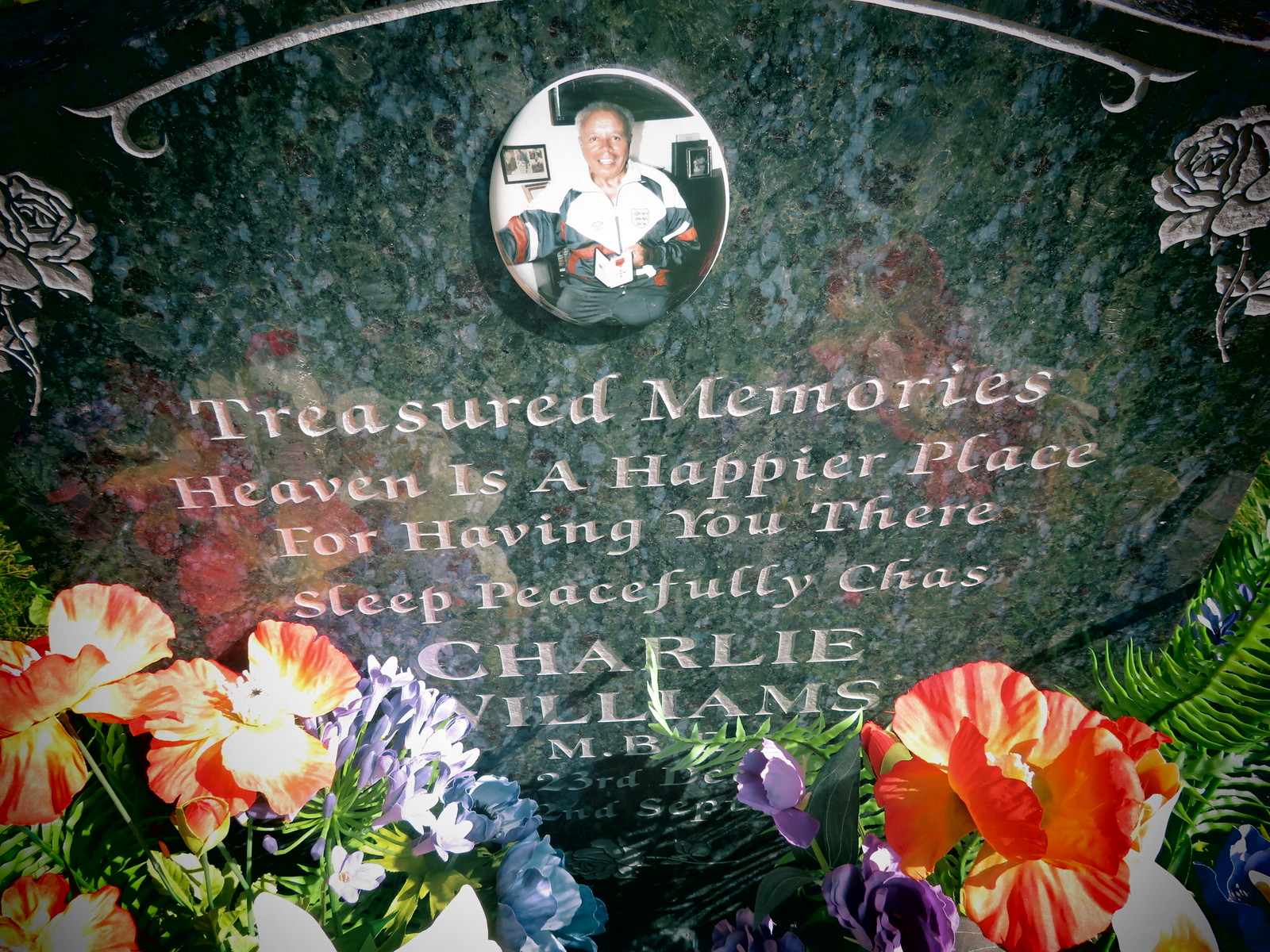This image vividly captures a granite headstone dedicated to Chaz Charlie Williams, engraved with the heartfelt inscription: "Treasured memories. Heaven is a happier place for having you there. Sleep peacefully, Chaz Charlie Williams." At the top of the headstone, there's an oval photograph of a smiling Charlie, possibly dressed in a jogging suit. The granite is a mottled blend of blue, green, gray, and black hues, adorned with intricately carved roses on either side of the picture. Surrounding the base of the headstone are vibrant flowers in shades of orange, purple, and white, mingled with green ferns. The flowers are abundant, covering the left and right corners and adding to the serene ambiance. The scene appears to be either in the evening or in low light, suggesting a peaceful, somber mood, though some shadows indicate the presence of a subtle light source. Near the bottom of the marker, partially obscured by flowers, are the numbers "23rd" and "second."